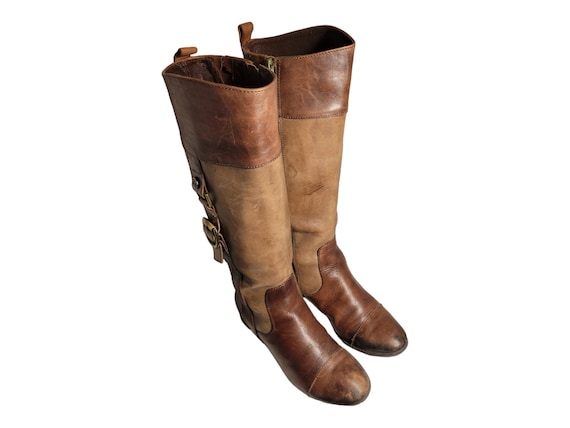This is a detailed photograph of a pair of knee-high cowboy boots against a white background. The boots, positioned diagonally facing the bottom right, showcase a distinctive mix of textures and colors. The lower portion, including the foot and heel area, is crafted from dark, shiny brown leather. This transitions into a worn-in, light brown suede material that covers from the ankle up to just below the knee. At the top, the boots feature a band of dark brown leather, similar to the bottom section, with a three to four inch cuff. Notably, each boot has a tab at the top for ease of pulling them on, and a tan-colored buckle is present on the right side of the right boot, adding both a functional and decorative element. The contrasting materials and colors create a visually appealing and practical design, potentially making these boots a standout item for sale or in a magazine feature.